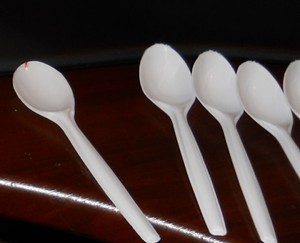In this photograph, five white plastic spoons are laid out on a mahogany brown tabletop. Four of the spoons are arranged close together in a row towards the center right of the image, while the fifth spoon is positioned a few inches apart from the others. This isolated spoon has a noticeable red spot on its tip, around the scooping edge. All the spoons are clean and aligned with their handles pointing downwards. A prominent white line, possibly a reflection of light, stretches from the lower left corner to the middle of the bottom edge of the photograph. The scene is illuminated by light coming from the left, enhancing the overall clarity and detail of the image.